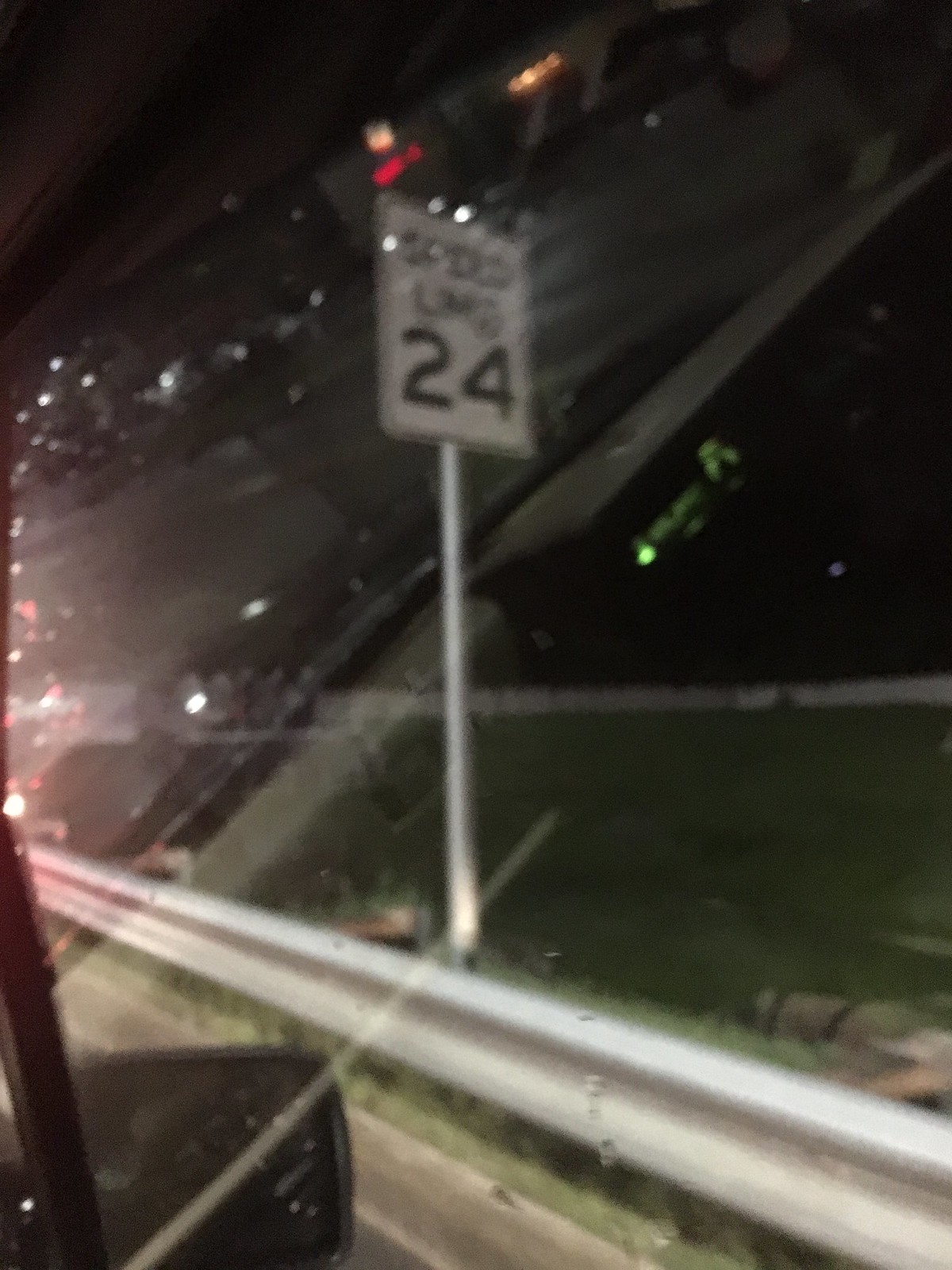This color photograph offers a unique perspective from the vantage point of a car window, capturing the essence of nighttime travel. Towards the foreground, the side mirror of the car is distinctly visible, reflecting the dim glow of the surrounding street lights. Diagonally cutting across the window from left to right is the reflection on the glass, creating an abstract pattern of light. On the roadside, a guardrail runs parallel to the car, providing a sense of motion and direction. In the mid-ground, a somewhat blurry speed limit sign reading "24" is poised against a green area on a black background, adding an element of mystery as the text is somewhat out of focus. The background is obscured in darkness, leaving much to the imagination. The upper section of the image features faint neon lights or signs, whose details are indistinct, adding a splash of color and urban allure to the scene. This intriguing photograph is a blend of reflections and ambient light, perfectly capturing the fleeting moments of a nocturnal drive.